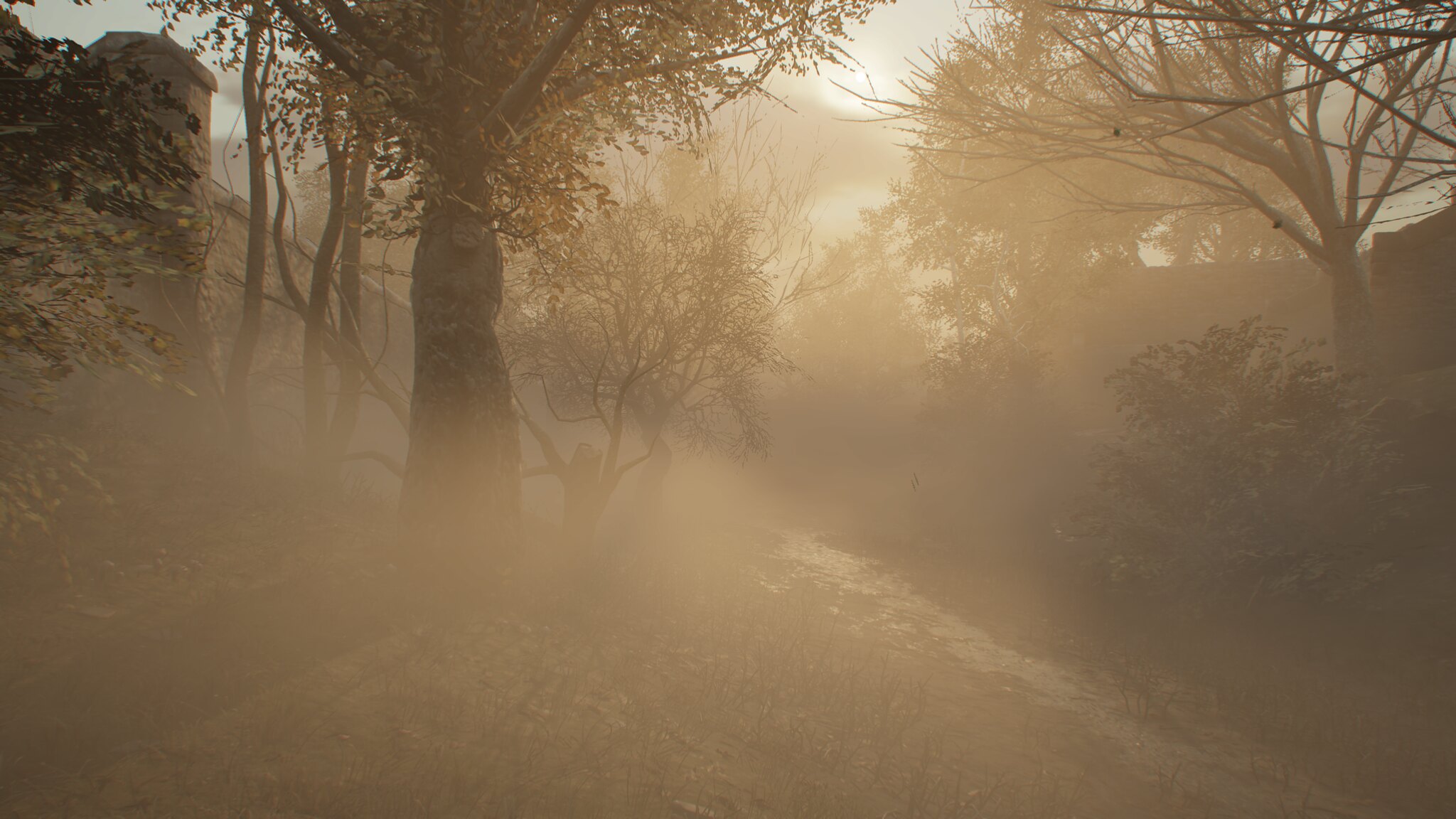In this detailed picture of a foggy valley, shrouded in a greenish-brown tint reminiscent of sepia tones, the scene is obscured by a dense haze giving it a surreal or possibly even digitally rendered appearance. On the right-hand side, a leafless tree stands tall beside a smaller bush, while further on, taller trees with scattered leaves add layers to the composition. A large deciduous tree dominates the area with what look like dead leaves, and surrounding it are three other tree trunks, along with a smaller trunk bearing a few dead branches. To the left, another fall-time tree retains some of its orange leaves, while the ground below is strewn with fallen leaves and dead branches. A small stream meanders diagonally from the right-hand corner toward the center, adding a dynamic element to the stillness of the scene.

A partially visible building emerges through the fog on the right, about three-quarters up the frame, hinted at by a level line and creating an eerie, obscured landmark. Another distant structure, possibly a wall or a turret, is barely discernible through the thick fog. In the background, the faint outline of hills suggests a mountainous setting, with the fog blending the horizon into a gray, ominous sky, enhancing the spooky atmosphere. A narrow trail is visible between the two foreground trees, but it vanishes into the misty distance, adding to the mysterious and ghostly feel of the image.